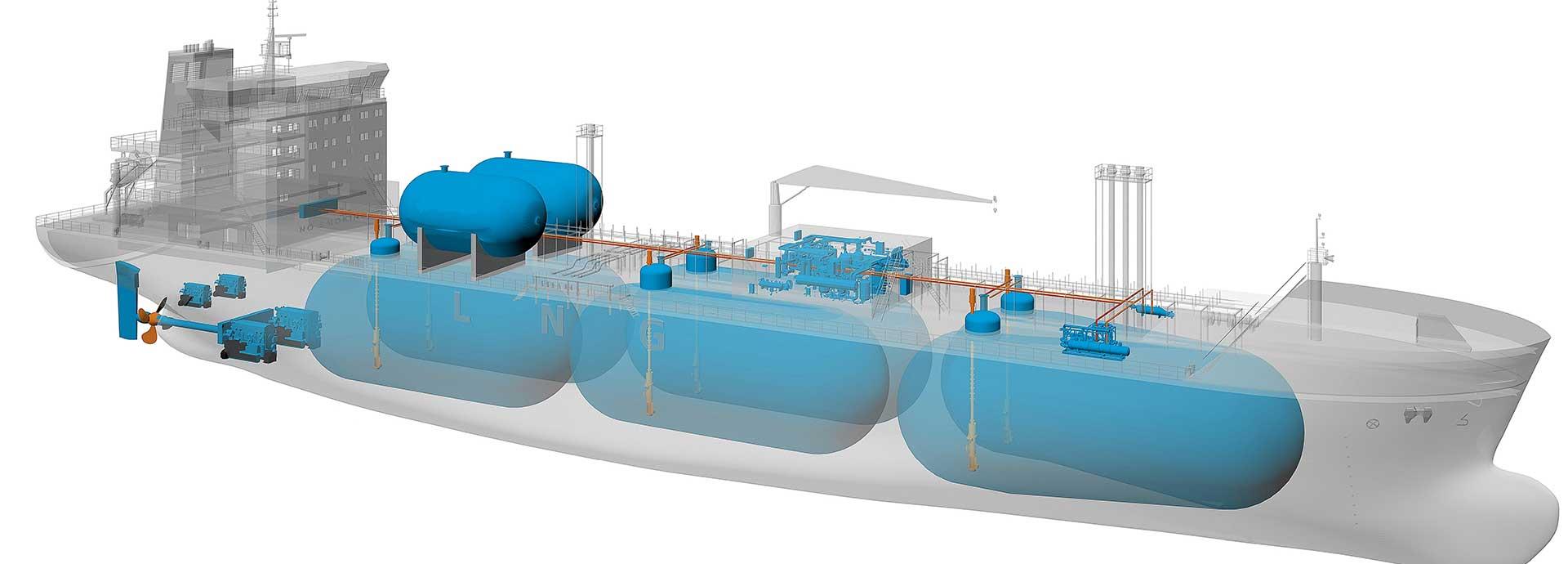The image showcases a detailed, see-through schematic of a large naval or industrial ship rendered in light gray to reveal its internal compartments. Centrally featured is a large, opaque gray building located near the stern, topped with a radar array and lined with windows. Stairs and scaffolding are adjacent to the building, providing access to various levels. Beside the building, two substantial blue holding tanks lay horizontally, followed closely by additional cylindrical tanks and manholes. These cylindrical manholes are systematically distributed along the ship's length, linked to more holding tanks, continuing toward the bow.

Inside the ship's hold, beyond the initial large holding tanks, two significant blue motors are connected to the ship’s propeller and a large fan. Two smaller motors are placed directly to the left of the large building. Gracefully rising from the bow is a stack of gray pipes. On the ship’s deck, two smaller oblong blue containers are conspicuously similar to residential natural gas storage units, held up by metallic structures. The focus on the blue interior barrels, resembling large oil or water containers, dominates the underdeck area with six substantial units depicted. The ship’s propeller, distinctively orange, highlights the stern's machinery area, standing out against the gray and blue hues of the vessel's intricate internals.